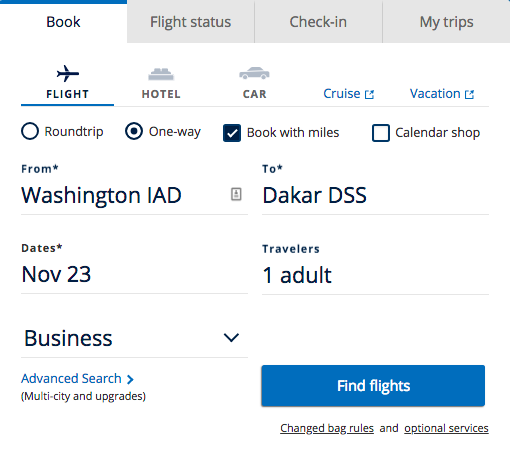The screenshot depicts a booking interface from a travel website. At the top, there are tabs for "Book," "Flight Status," "Check-In," and "My Trips." The "Book" tab is selected, highlighted in white with a blue bar, while the other tabs have a gray background. Below this, there are options for booking a flight, hotel, or car, indicated by icons of an airplane, a building, and a car, respectively. Additionally, there are pop-up options for booking a cruise or a vacation.

Currently, the "Flight" option is selected, as denoted by the black text underlined in blue. The user has chosen a "One-way" flight, indicated by the selected radio button. They have also selected the option "Book with Miles." The travel details specified are from Washington Dulles International Airport (IAD) to Blaise Diagne International Airport in Dakar (DSS), with the departure date set for November 23rd. The booking is for one adult traveling in business class, which suggests a significant expense.

Additional options such as "Advanced Search," "Multi-City," and "Upgrades" are available but not selected. A prominent blue button labeled "Find Flights" awaits to be clicked. Below this button, there is a link for "Changed bag rules and optional services." Given the route and class, it is anticipated that this one-way ticket from Washington to Dakar will be costly. Good luck to the traveler, especially in securing an affordable fare in business class.